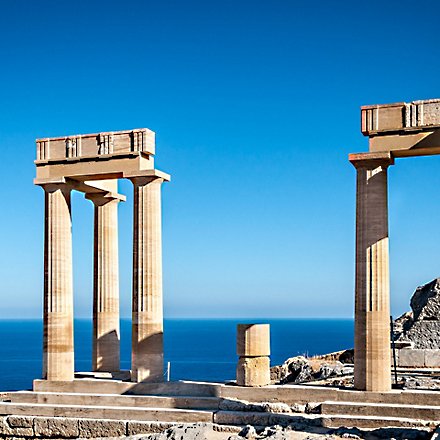The image depicts ancient Roman ruins, featuring several monumental columns situated near the sea. The ruins are primarily composed of tall columns with minimal remnants of the original structure atop them. Notably, three colossal columns, possibly 50-80 feet in height, remain standing together, while one nearby column lies mostly toppled, retaining only its bottom portion erect. These ruins rest on a small staircase or podium, giving an elevated perspective that suggests a hill or mountain setting. The backdrop presents a visually stunning, calm, and expansive sea of deep blue, seamlessly merging with an equally clear sky that fades from a lighter blue at the horizon to a darker blue as it ascends. The overall scene is captured on a bright, sunny day, accentuating the timeless and serene atmosphere of these majestic ancient ruins.